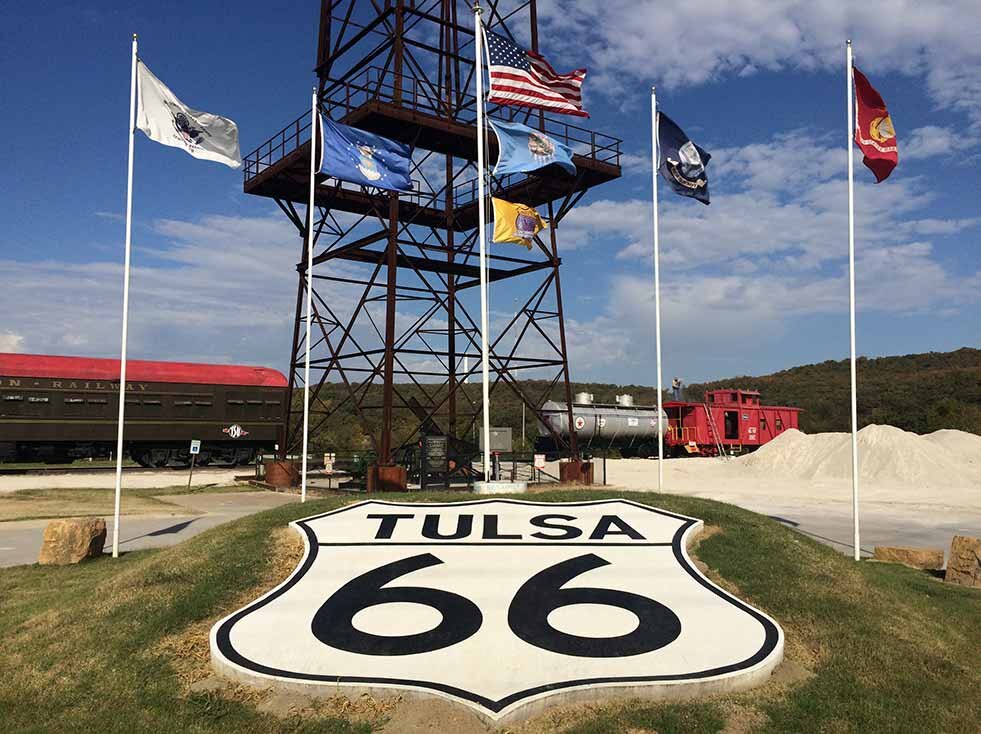The image captures a scenic but detailed stop along the legendary Route 66 in Tulsa, Oklahoma. In the foreground, a large highway sign stands prominently on a small grassy hill, shaped like a badge and divided into two parts. The top part is labeled "Tulsa," and the bottom part features the number "66." Surrounding the sign in a half-arch formation are several flags, with the tallest being the United States flag, accompanied by various others including a white flag, a blue flag with a white emblem, a navy blue flag with an emblem and banner, and a red flag with a similar design.

In the background, a railway stretches out with tracks running parallel to green hills and mountains. On the left side of the image, a black train car with a red roof partially extends out of the frame, followed by a silver tanker car designed to carry liquid, and then a standard red cargo car. A large, towering radio or observation tower rises between the camera and the train tracks, featuring a small platform about 20 feet up, equipped with guardrails. The sky above is blue, adorned with scattered clouds, giving a picturesque backdrop to this slice of American nostalgia.